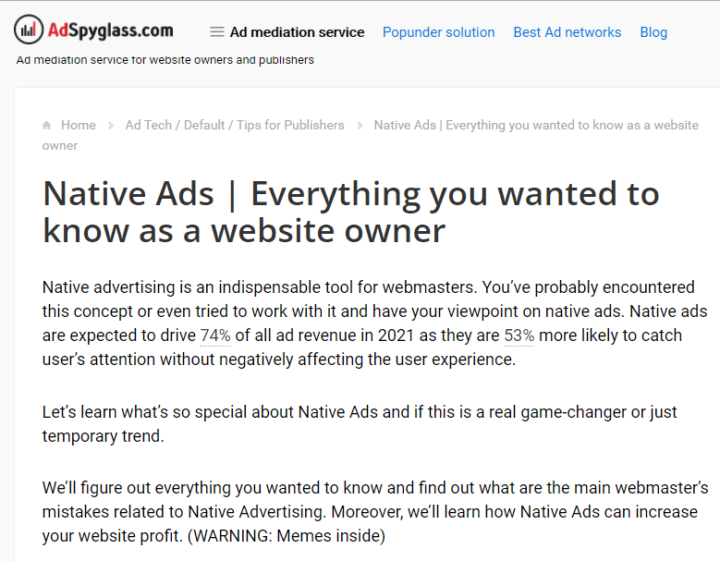The screenshot depicts the homepage of a website, iSpyGlass.com. The layout features distinct sections that include "Ad Mediation Service," "Ponder Solution," "Best Ad Networks," and "Blog." These sections are highlighted in blue, indicating that they are clickable links for more information.

In the lower section of the webpage, a prominent black heading states, "Native Ads: Everything You Wanted to Know as a Website Owner." This area provides an in-depth overview of native advertising's importance for website owners. The text explains that native advertising is a vital tool for webmasters, likely familiar to them either through firsthand use or general awareness. The passage highlights the impact of native ads, noting that they are projected to generate 74% of all ad revenue in 2021 by being 53% more effective at capturing users' attention without detracting from the user experience.

Further, the content promises to demystify native ads, exploring their potential as either a significant innovation or a fleeting trend. The section aims to address common mistakes made by webmasters when dealing with native advertising and to demonstrate how native ads can boost website profitability.

At the bottom, the text includes a playful warning: "Memes inside." The overall design of the page features a clean white background with black text, complemented by the website’s logo—a circular graphic illustrating mostly black bar graphs with the final bar in red. The visual elements and detailed content work together to convey a professional yet engaging atmosphere, inviting users to explore the topic further.